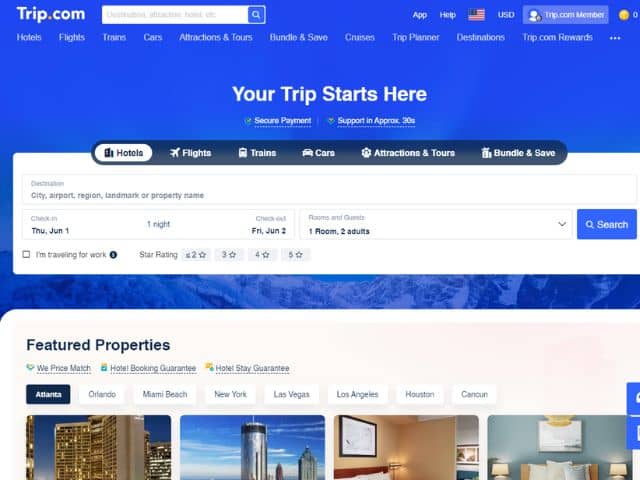**Detailed Caption:**

The web page features a dark blue header positioned at the top left, prominently displaying the logo "trip.com" in bold white text with an orange dot separating “trip” and “com”. Below the header, there is a search bar with indistinct gray text and a search icon represented by a white magnifying glass within a dark blue square. 

On the right side of the header, there are several clickable sections that include "App", "Help", an American flag indicating language preferences, and "USD" suggesting currency selection. Adjacent to these, a lighter blue rectangle contains a silhouette of a person, symbolizing a user profile, which displays "trip.com" and "Remember Me". Below this, a blurred profile face icon accompanied by a zero probably indicates the current user's profile status or points.

The navigation bar below the header features multiple clickable tabs: "Hotels," "Flights," "Trains," "Cars," "Attractions," "Tours Bundle and Save," "Cruises," "Trip Planner," "Destinations," and "trip.com Rewards". An ellipsis suggests more options.

Highlighted prominently in bold white text are the words "Your Trip Starts Here", positioned beneath the navigation bar. Alongside this phrase, a green shield with a checkmark indicates "Secure Payment", followed by an ellipse. Another ellipse follows the phrase "Support in approximately 30 seconds".

Below the header and navigation bar, a new black oval section with clickable buttons is visible. The first button is highlighted, changing from black to white, and displaying an icon of black buildings with the text "Hotels". Subsequent icons and their respective labels include a plane ("Flights"), a train ("Trains"), a car ("Cars"), a group of people ("Attractions"), and a combined icon for "Bundle and Save" featuring a hotel and a cruise.

Further down, a light gray rectangle titled "Destination" includes a note, "city, airport, region, landmark, or property name" as the place to enter search specifics. 

Another section displays a check-in feature within a rectangle. The check-in date is presented in bold with the day abbreviated as "THU" (Thursday), the month as "JUN" (June), and specifies a one-night stay. The check-out date follows, marked as "Friday, June 2nd". Additionally, the section details the number of rooms and guests, exemplified by "1 room, 2 adults". 

A search button is present, and beneath this, a "Feature Properties" section showcases images of various buildings: a brown building, a silver building, a tan building, and a group of buildings.